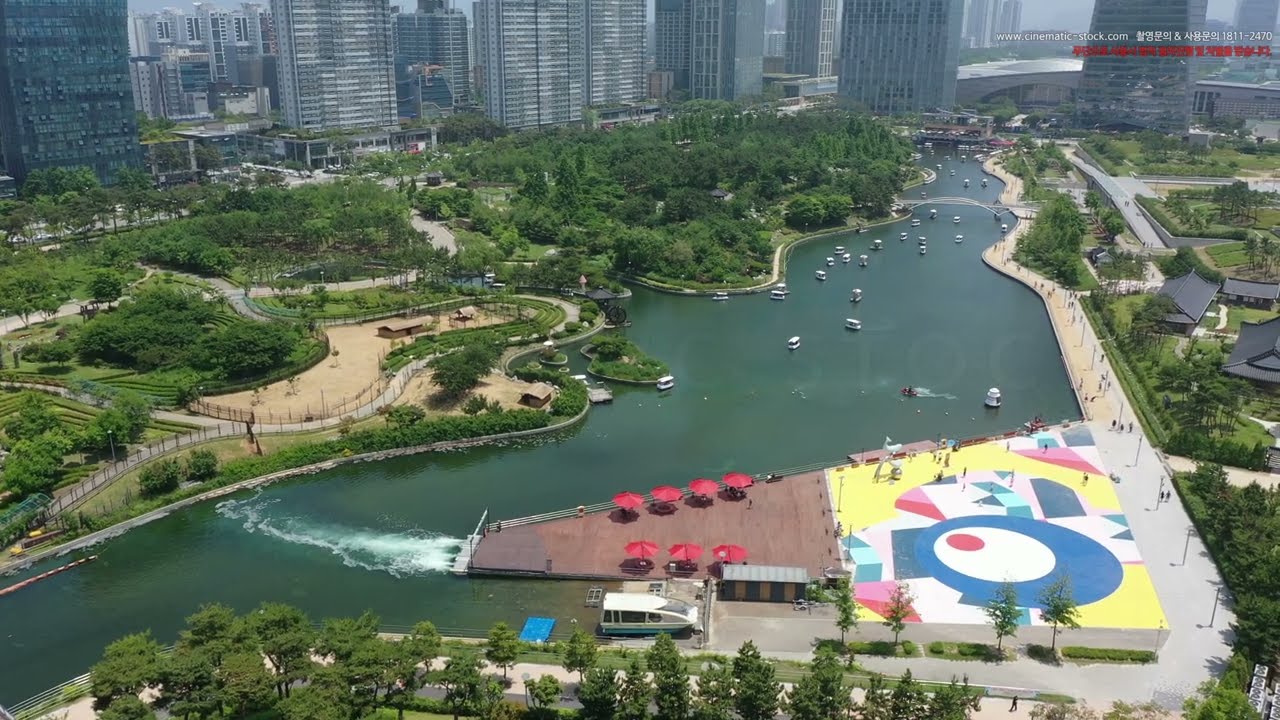The image is a color landscape aerial photograph capturing an urban river scene, likely taken by a drone. In the background, a row of towering gray commercial high-rise buildings with numerous windows suggests it is a large city, potentially in China or Japan, indicated by the mandarin script and a red font URL in the top right corner (www.cinematicstock.com). The sky appears gray and foggy, contributing to the city's bustling ambiance. 

The river runs through the center of the image, populated with various recreational paddle boats and love boats. On the right side of the river, a long sidewalk bustling with pedestrians leads to a vibrant gathering space adorned with a colorful geometric art display featuring rainbow colors and a distinct white and blue bullseye pattern. This area is adjacent to a triangular deck with seven red umbrellas, likely for dining and drinking, and a docking area for boats. Scattered throughout the scene are patches of greenery, including trees and grass, adding a touch of nature to the urban landscape.